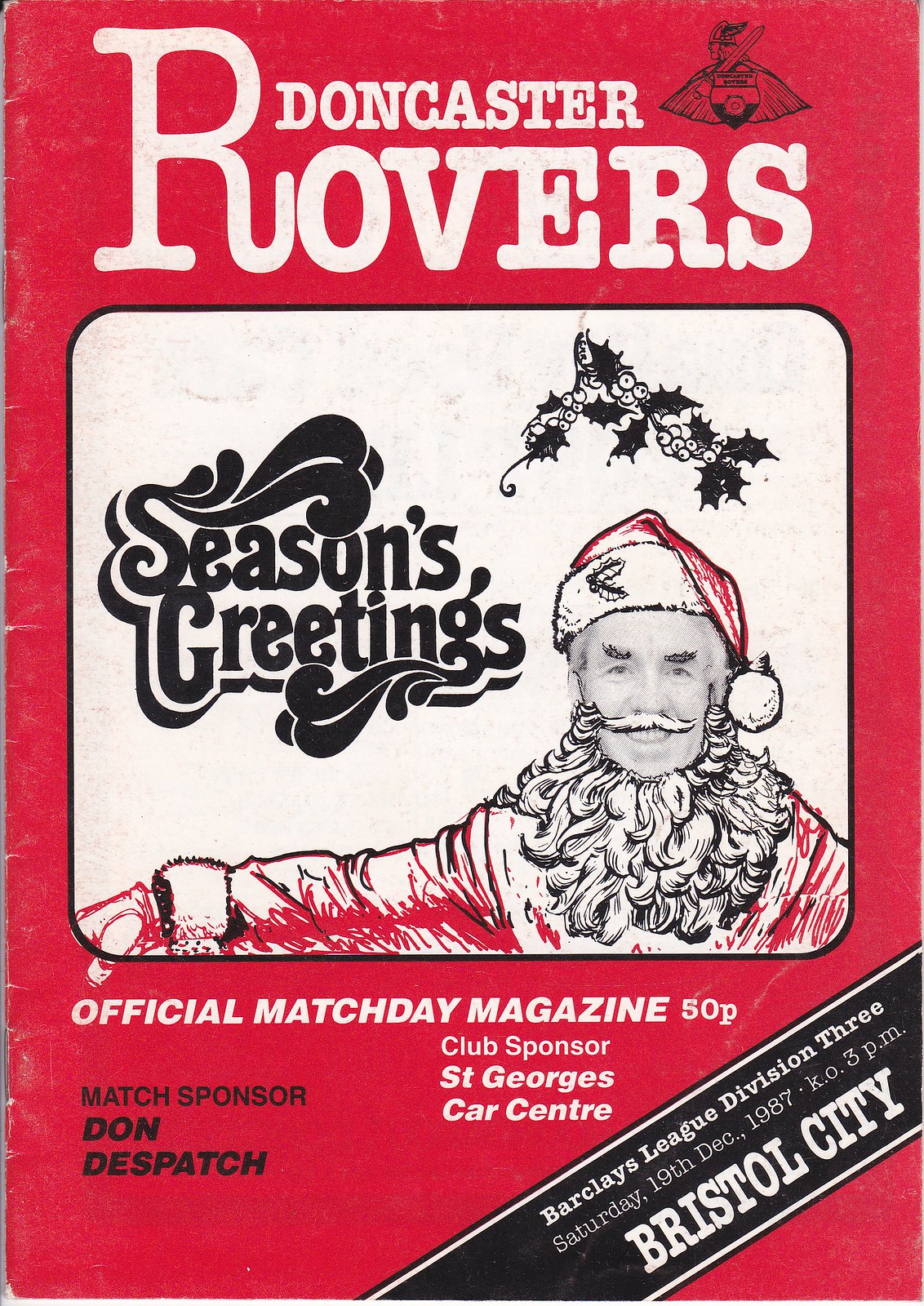The cover of the Official Match Day Magazine for Doncaster Rovers features a festive design with a red background and white text at the top reading "Doncaster Rovers." Central to the cover is a humorous, festive image of a Santa Claus, with the face of someone likely affiliated with the football club, dressed in a traditional Santa outfit complete with a big beard and a cheerful smile. Above Santa's head are black poinsettia leaves, and adjacent to him, in black text, it reads "Season's Greetings." In the top right corner of the cover, there is a small black insignia depicting a Viking with a sword and shield. Below the festive imagery, the magazine denotes its purpose and price: "Official Match Day Magazine, 50p." Further details include the club's sponsor, St. George's Car Center, and the match sponsor, Dawn Dispatch. The bottom right corner, framed with a black border, details the match information: "Barclays League Division III, Saturday 19th December 1987, KO 3 pm, Bristol City."